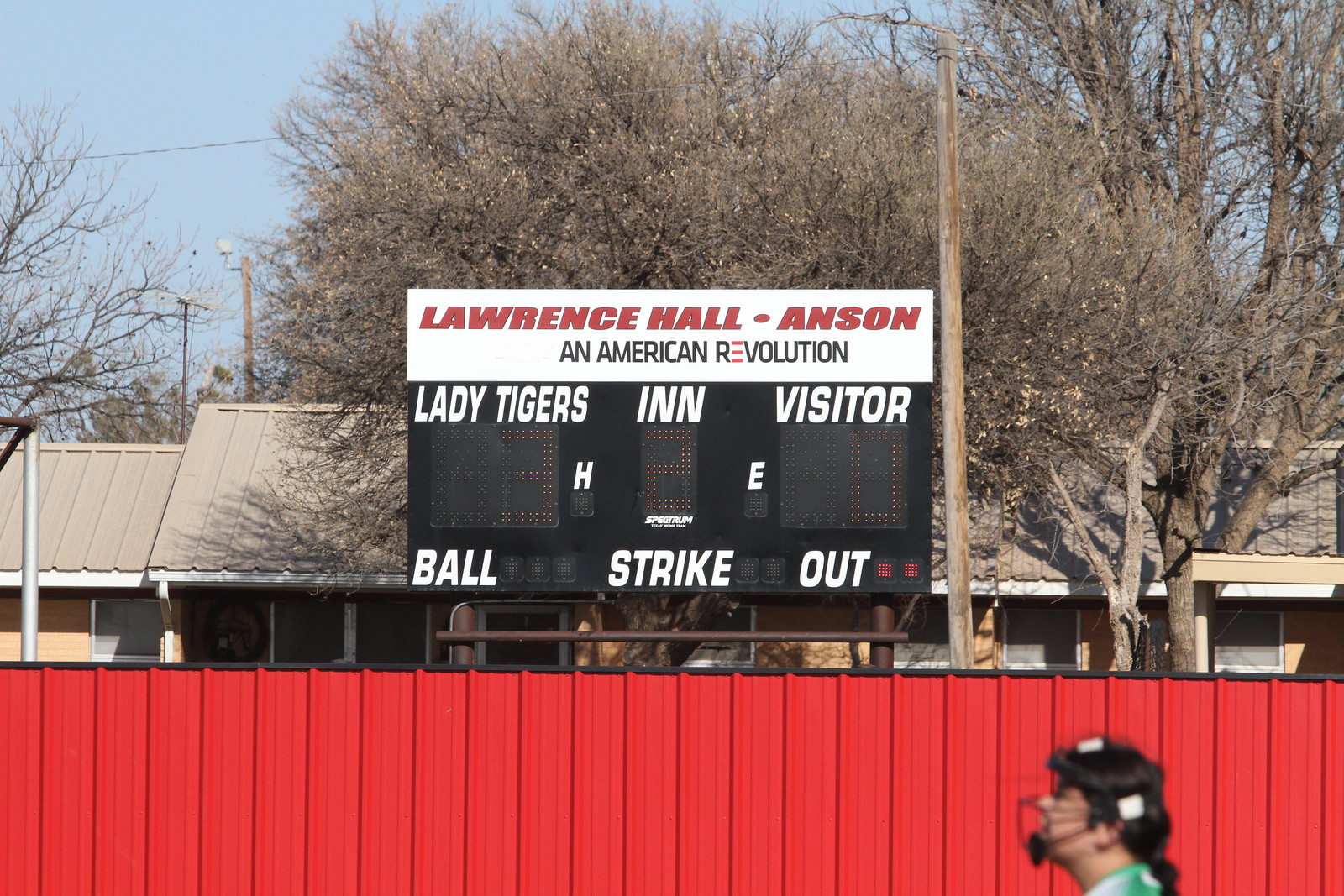The image depicts a baseball scoreboard prominently situated behind a red fence with vertical planks. The scoreboard is supported by two vertical poles with a connecting horizontal pole at the top. The top of the scoreboard features a white border with the text "Lawrence Hall-Anson" in red letters, followed by "An American Revolution" underneath. The main scoreboard interface shows "Lady Tigers" in white on the left and "Visitor" on the right, separated by "INN" (inning) in the middle. Below "Lady Tigers," there's "3" indicating their score, and below "Visitor," there's "0" for their score. Under the "3" for Lady Tigers is an "H," and under the "0" for Visitor is an "E." The inning is displayed as "2." The bottom of the scoreboard has sections labeled "BALL," "STRIKE," and "OUT" in white letters, with no lights illuminated for "BALL" or "STRIKE," but two lights lit for "OUT." To the bottom right corner of the scoreboard, partially obscured by the fence, is the head of a person wearing an umpire's helmet with a wire face mask, looking to the left. In the background, there is a building and some leafless trees, suggesting a colder time of year and creating a somewhat gloomy atmosphere.